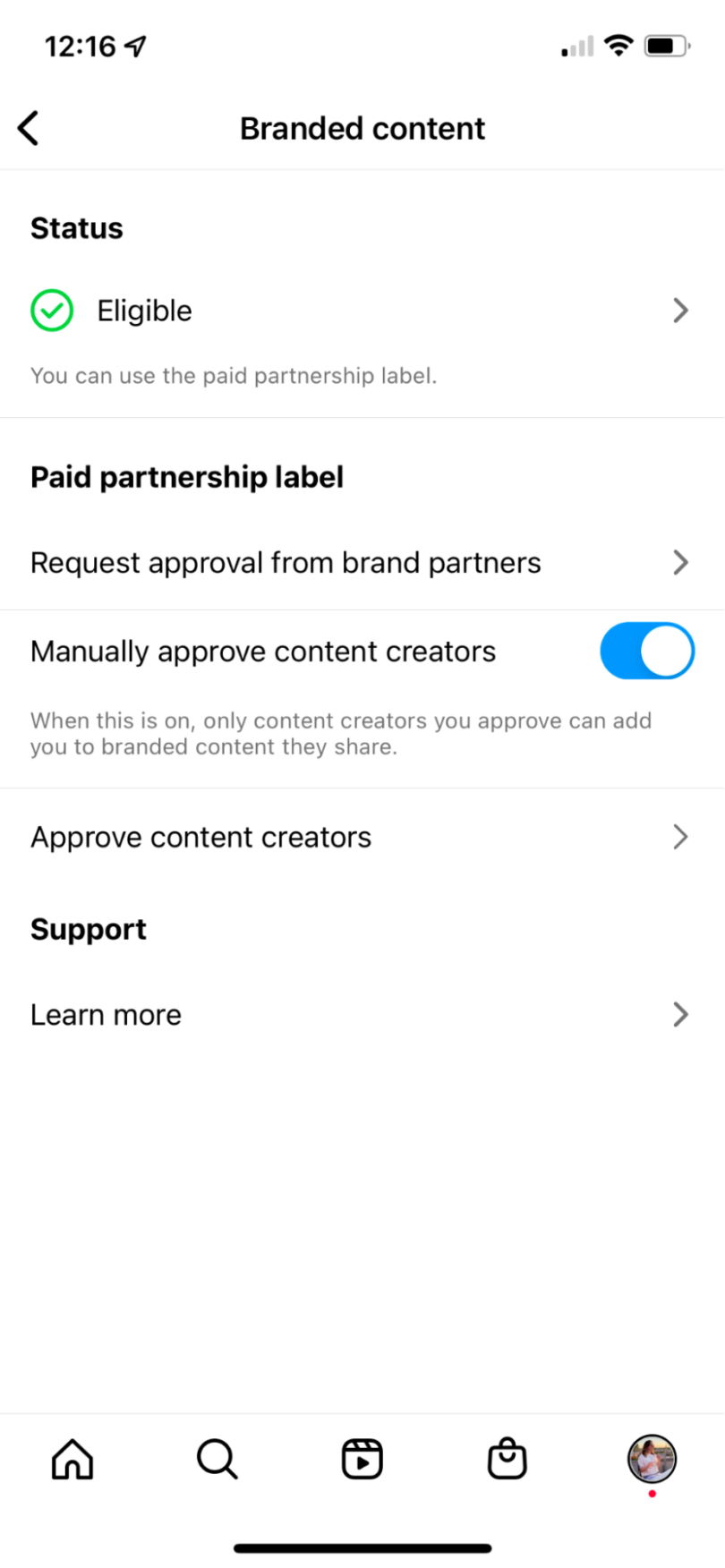The image is a screenshot from a mobile device captured at 12:16. The status bar indicates that location services are enabled, the carrier signal is at one bar, Wi-Fi is at full strength, and the battery is approximately 70% charged. Central to the screenshot is a user interface related to branded content settings. At the top-left corner, there is a back arrow in black. Below this, the title "Branded Content" is displayed in black font. The main section shows a green circle with a green checkmark and the word "Eligible" in black. There is an "Open" option suggesting that the user can utilize the paid partnership label.

Further down, additional options include "Paid Partnership Label," "Request Approval from Brand Partners," and another "Open" option, which presumably expands these settings. There is also a toggle switch, shown in blue as enabled, with text explaining its function: "When this is on, only contact creators you approve can add you to the branded content they share." The text appears twice, possibly due to a glitch or redundancy.